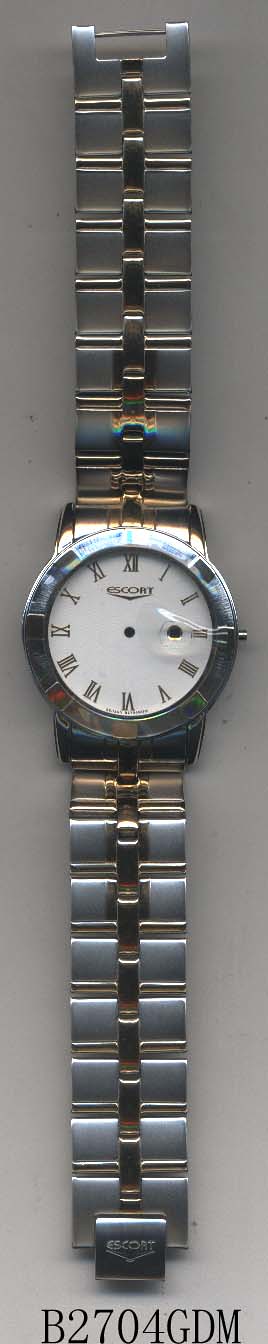This vertical photograph showcases an elegant wristwatch, featuring a distinctive silver-gold link band that exudes a masculine appearance due to its robust design. The watchband is crafted with alternating silver rectangular links, connected by vertical interlinks, adding to its sophistication. The watch's case is fashioned from a platinum-like silver metal, contributing to its polished and refined aesthetic.

The dial of the watch is a clean white, adorned with black Roman numerals, though it is noteworthy that the hands of the watch are absent. The timepiece is a product of the brand Escort, as evidenced by the branding stamped on the clasp of the band, which secures it to the wrist.

At the bottom of the image, there is a prominent model number written in large, bold, black lettering: B2704GDM. This detail highlights the specific model of the watch, adding an element of identification and uniqueness to the photograph.